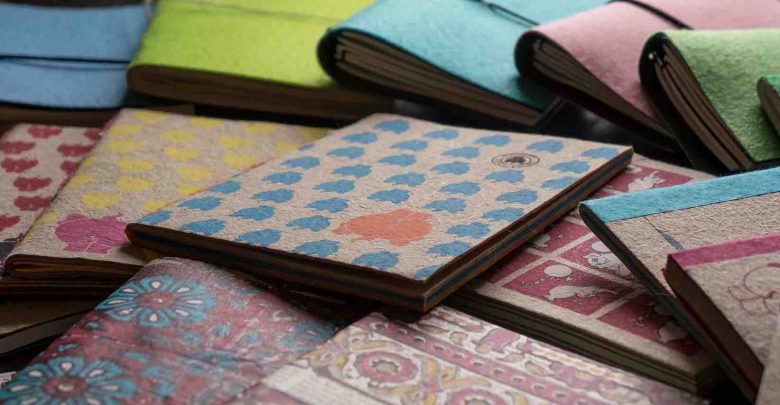This close-up image showcases nearly ten upcycled craft projects, which appear to be small notebooks, journals, or organizers. They are made of recycled materials and are meticulously arranged in a fanned-out and somewhat random pattern. 

In the back row, there are several felt-covered journals in solid colors: light blue, green, light green, purple, and dark green. Most of these are slightly cut off in the photograph. Moving to the middle and front rows, there are brown paper notebooks adorned with vibrant designs and patterns. These notebooks feature a variety of patterns, including beige with blue and orange, beige with red and yellow, beige with red, green, maroon, and a paisley floral design. 

Specific details include notebooks with red and turquoise blue flower designs, red square stamps, blue dots with a pink splotch, rings of blue abstract patterns repeated across one cover, red butterflies, yellow butterflies, and solid blue and green covers. There are also a couple of notebooks with light blue spines and one with a medium shade pink spine.

Overall, the image captures the creativity and diversity of these handmade, eco-friendly products, highlighting the textures, colors, and artistic details that make each one unique.